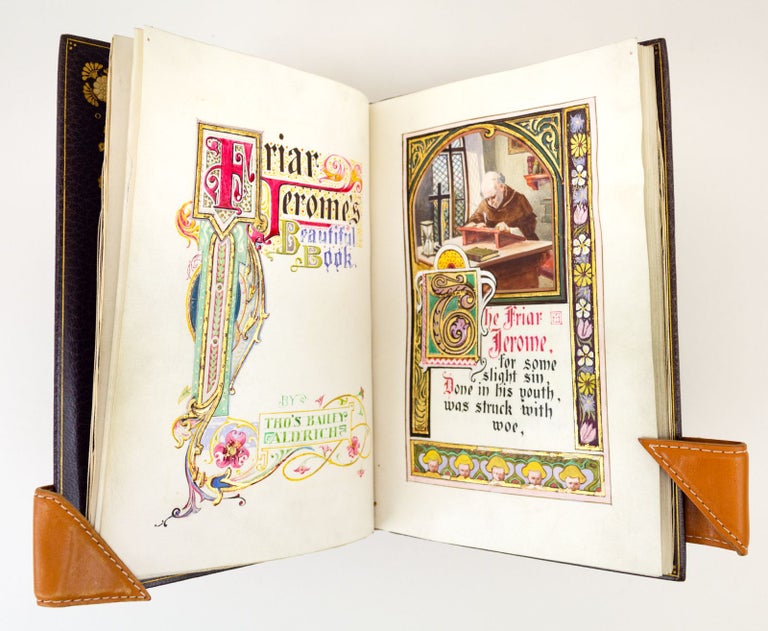This photograph features an ornate, leather-bound book displayed upright on a white background, supported by brown leather straps at the bottom corners to hold its pages open. The left page, adorned with lavish designs including pink flowers and yellow gold curlicues, bears the title "Friar Jerome's Beautiful Book" in an Old English style with an ornate, large capital "F" from which intricate scrollwork with floral elements extends. Beneath the title, in green text that is too small to read, the author is identified as Aldrich or Galdric. The right page showcases an illustration of a balding friar, presumably Friar Jerome, dressed in a black cape and gown, seated at a table with a tilted reading stand. He appears to be in a church, indicated by the presence of a cross and stained glass windows in the background. Underneath the illustration, a passage reads, "For some slight sin done in his youth, was struck with woe." The pages are bordered by detailed, flowery patterns, enhancing the antique and artistic aesthetic of the book.